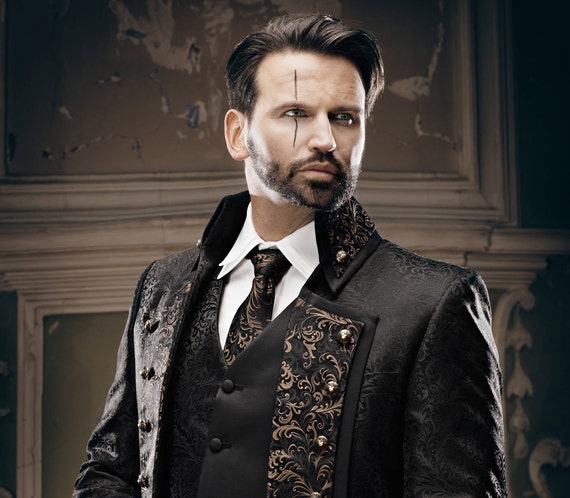The image features a man in a three-piece black suit adorned with intricate golden floral designs on the jacket, vest, and tie, which exudes an air of ornate sophistication, reminiscent of an Indian wedding outfit. His hair, short and slicked back, complements his well-groomed beard. A notable aspect of his appearance is a prominent scar that runs across his left eye, marked by two lines—one above and one below. He stands slightly angled to the left, with his head turned more toward the right, gazing into the distance. Underneath his elegantly designed suit, he wears a crisp white shirt. The background hints at a refined setting with grayish and beige tones and includes elements that suggest a fireplace or textured mantle, adding depth to the scene. The overall ambiance of the image is dark and subtly colored, possibly indicating an opulent, yet somber, environment.